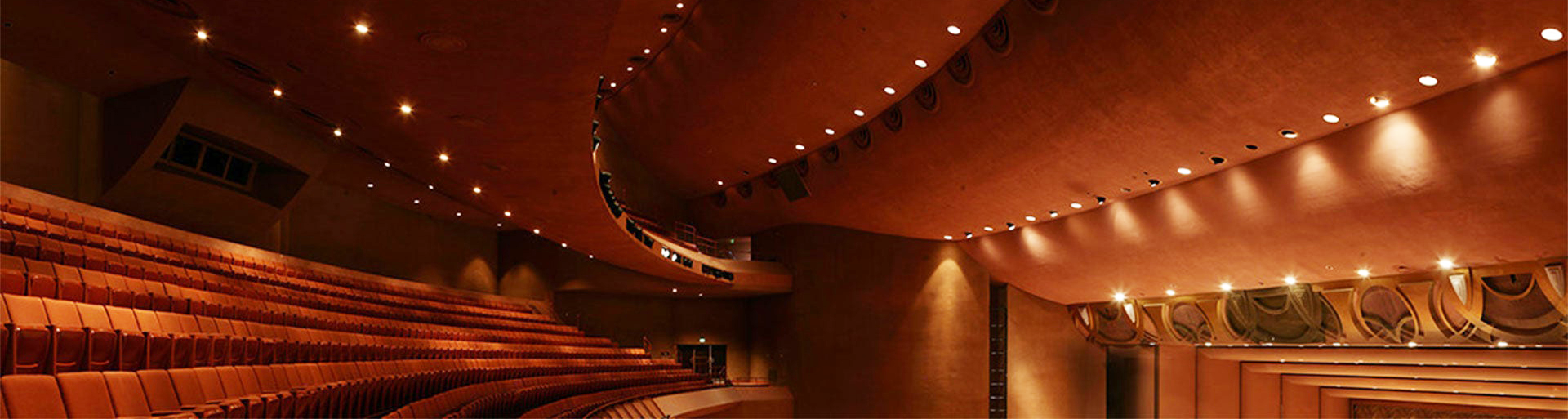The image captures the interior of a grand theater, presented in a wide, horizontally oriented rectangular frame. Dominated by a deep reddish-brown cast, the ceiling features a series of ridged, horizontally running panels, with each ridge adorned by a row of tiny, round white lights. These long burgundy panels create a layered effect, drawing the eye upward. Below, rows of empty seats in matching burgundy hue are visible. On the left side, the seating arrangement resembles stadium-style curved sections, likely part of the balcony seating. The right side hints at the top of the stage area, featuring intricate gold trim and ornate design patterns, further accentuating the theater's opulence. Light tan walls flank the seating, and additional architectural details, such as speakers and windows, are subtly integrated into the background.